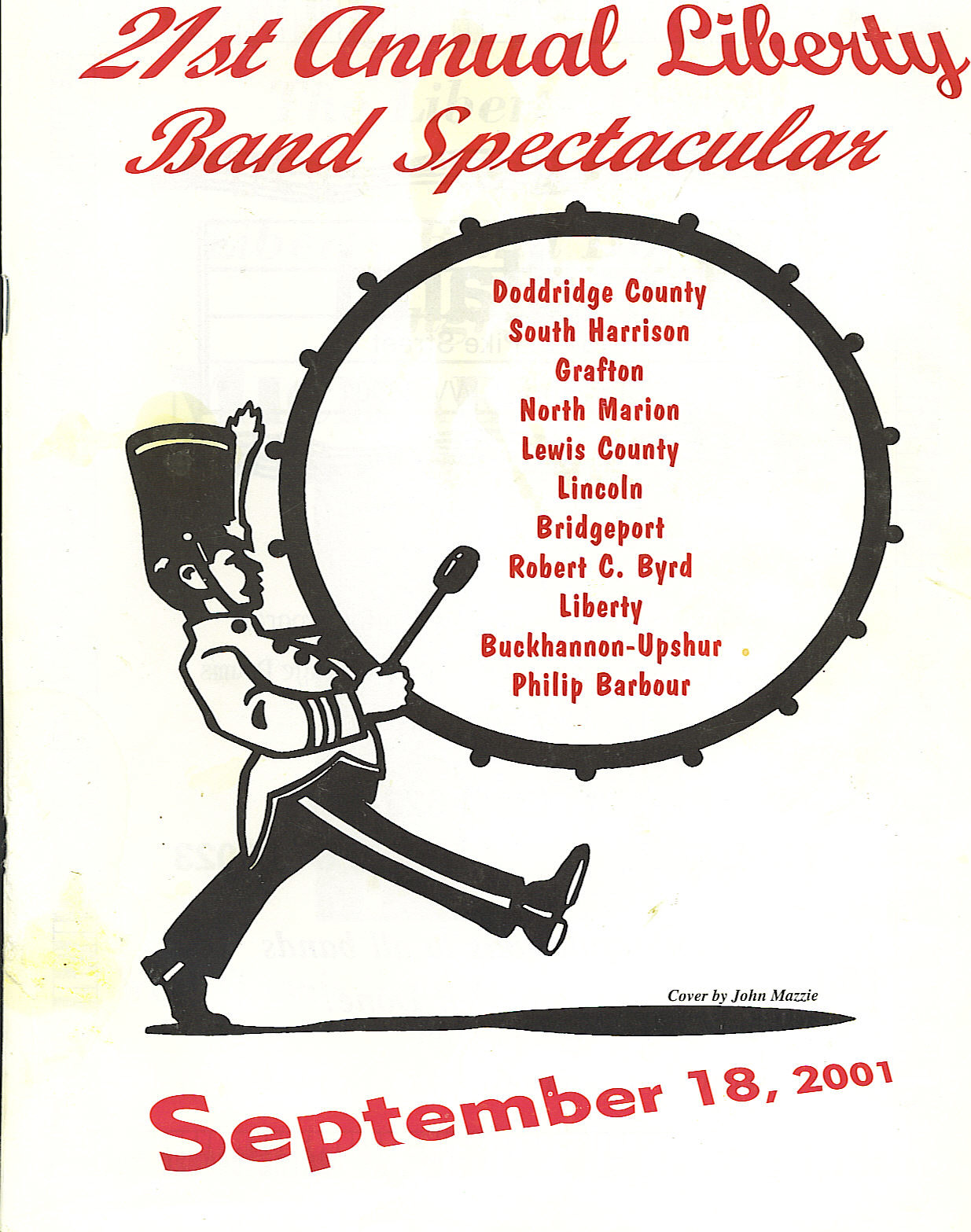This image depicts an old, discolored program cover for the 21st Annual Liberty Band Spectacular, held on September 18, 2001. The cover, now an off-white shade with pinkish stains, features a prominent graphic of a marching band member dressed in a tall hat, white jacket, and black pants with a stripe down the leg, carrying a large bass drum. The title "21st Annual Liberty Band Spectacular" is displayed at the top in bold, red cursive script, while the date "September 18, 2001" is written diagonally at the bottom, also in red. The bass drum graphic centrally lists various participating counties in red print, including Doddridge County, South Harrison, Grafton, North Marion, Lewis County, Lincoln, Bridgeport, Robert C. Byrd, Liberty, Buckhannon-Upshur, and Philip Barbour. Additionally, the bottom left corner credits the cover design to John Mazel. The left-hand side vertically shows a pinstripe and remnants of two staple marks, suggesting it was once part of a booklet.